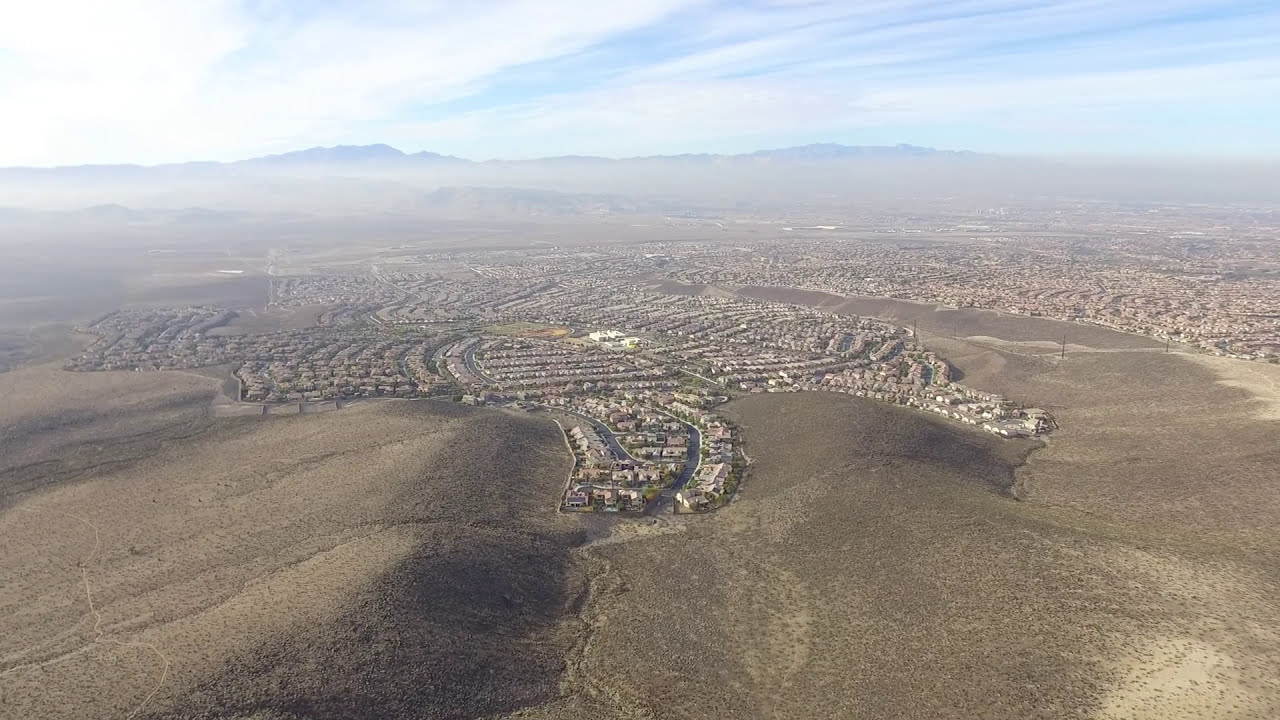This high-elevation image captures a vast desert landscape with a sprawling town at its center. The foreground features mostly flat, dark gray or brown desert terrain, devoid of any structures, which transitions into the town further in the distance. This town appears densely packed with rows of houses, characterized by their cookie-cutter uniformity. Prominently standing out among the residential areas is a distinctive property with white buildings, possibly a mansion or a commercial complex. The arid environment surrounding the town is predominantly brownish, suggestive of either sand or dried plants. As the landscape extends towards the horizon, it becomes increasingly hazy, eventually merging with distant shallow mountains. Above this scene, a clear sky is dotted with a few clouds, and the air carries a visible layer of dust, adding to the overall impression of dryness and heat.